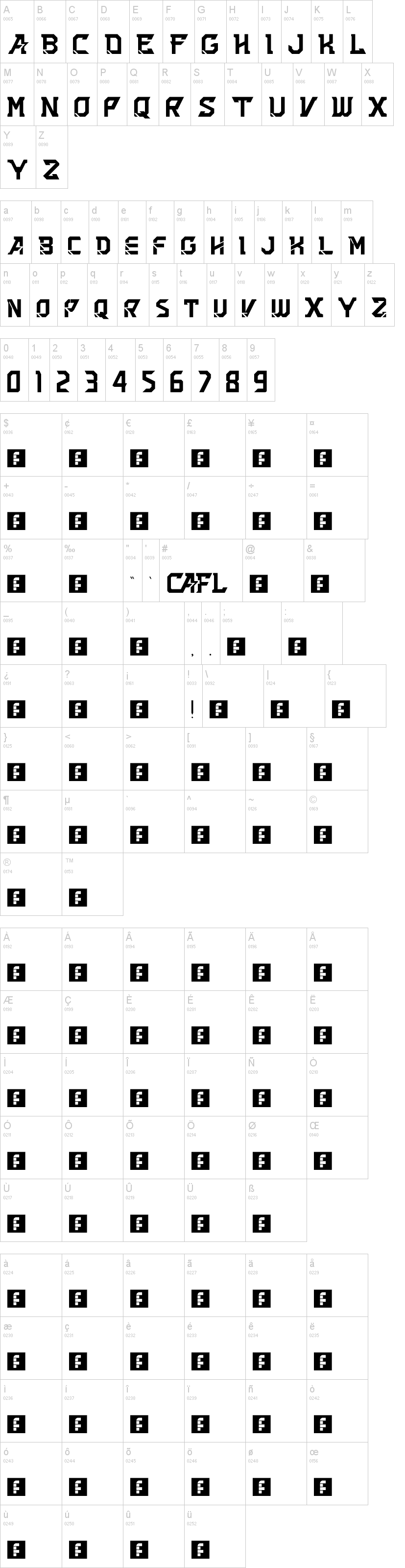The image depicts an organized grid of characters, numbers, and symbols, reminiscent of a keyboard layout. At the top, a row of twelve neatly arranged small boxes, each containing a single bold black letter, spans from left to right starting with 'A' and ending with 'L'. Below this, another row continues with letters 'M' through 'Z', each housed in its own box in the same bold format.

Proceeding downwards, the pattern repeats with a smaller version of the previous rows. The first row of this new section displays letters 'A' to 'M', and the subsequent row completes the alphabet with 'N' to 'Z', all in bold black letters within their respective boxes.

The next section showcases numeric characters, where each of the ten boxes contains a single bold black number from '0' to '9'. After the numbers, the image features multiple sections of black rectangles containing a bold white 'F'. The first group consists of six boxes across two rows, followed by a smaller set of two boxes flanking letters 'C', 'A', 'F', and 'L'.

Further down, there are configurations of five to six boxes per row, each with a white background and a black rectangle inside, displaying the bold white 'F'. These arrangements of boxes span several rows in different groupings - with transitions from two rows of six, to one row of two, multiple rows of six, and eventually narrowing to a single row of five boxes.

Near the bottom of the image, additional rows of six boxes precede the conclusion of five rows of six boxes each. The ultimate section showcases four black boxes on the lowest row, each featuring a bold white 'F' in the center. The overall structured design of this image, with its repetitive and regimented layout of characters, numbers, and symbols, resembles a highly organized keyboard template or data input grid.